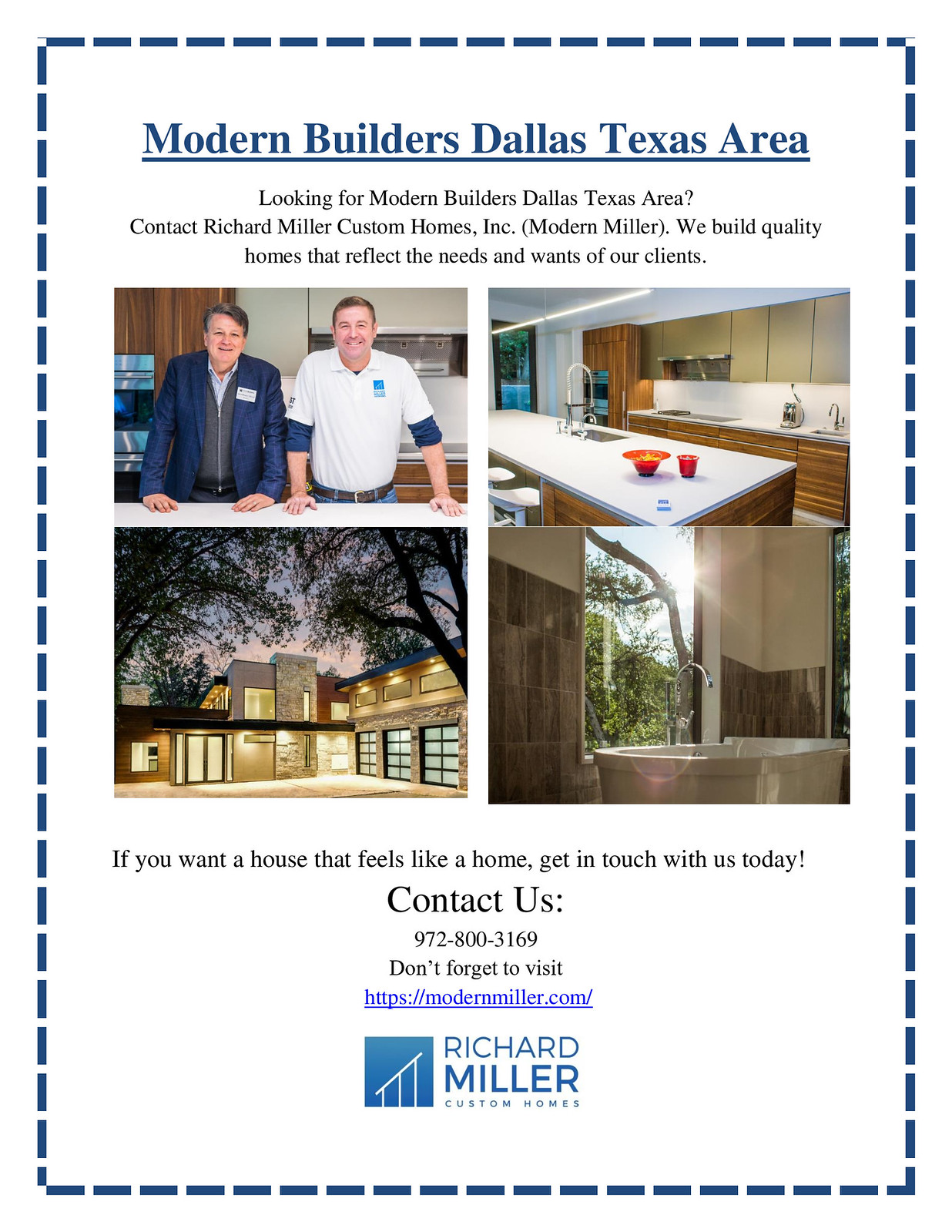The image is an advertisement for Modern Builders, situated in the Dallas, Texas area. The ad is framed with a dashed border, predominantly features blue and black text. At the top, bold blue text underlined in blue reads "Modern Builders, Dallas, Texas area." Below, in regular black text, it states, "Looking for Modern Builders in the Dallas, Texas area? Contact Richard Miller, Custom Homes Inc. (Modern Miller). We build quality homes that reflect the needs and wants of our clients."

Accompanying the text are four pictures: one of two men, one in a blue suit jacket and gray vest and the other in a white shirt with a blue long-sleeve shirt underneath, both touching a white table; a kitchen featuring white countertops with a central sink; a luxurious exterior of a house with lights on; and a bathroom with brown tile walls, a bathtub, and a sunlit exterior view through see-through windows. 

At the bottom, it states, "If you want a house that feels like a home, get in touch with us today," followed by contact information, a website in blue, and the Richard Miller Custom Homes logo also in blue.